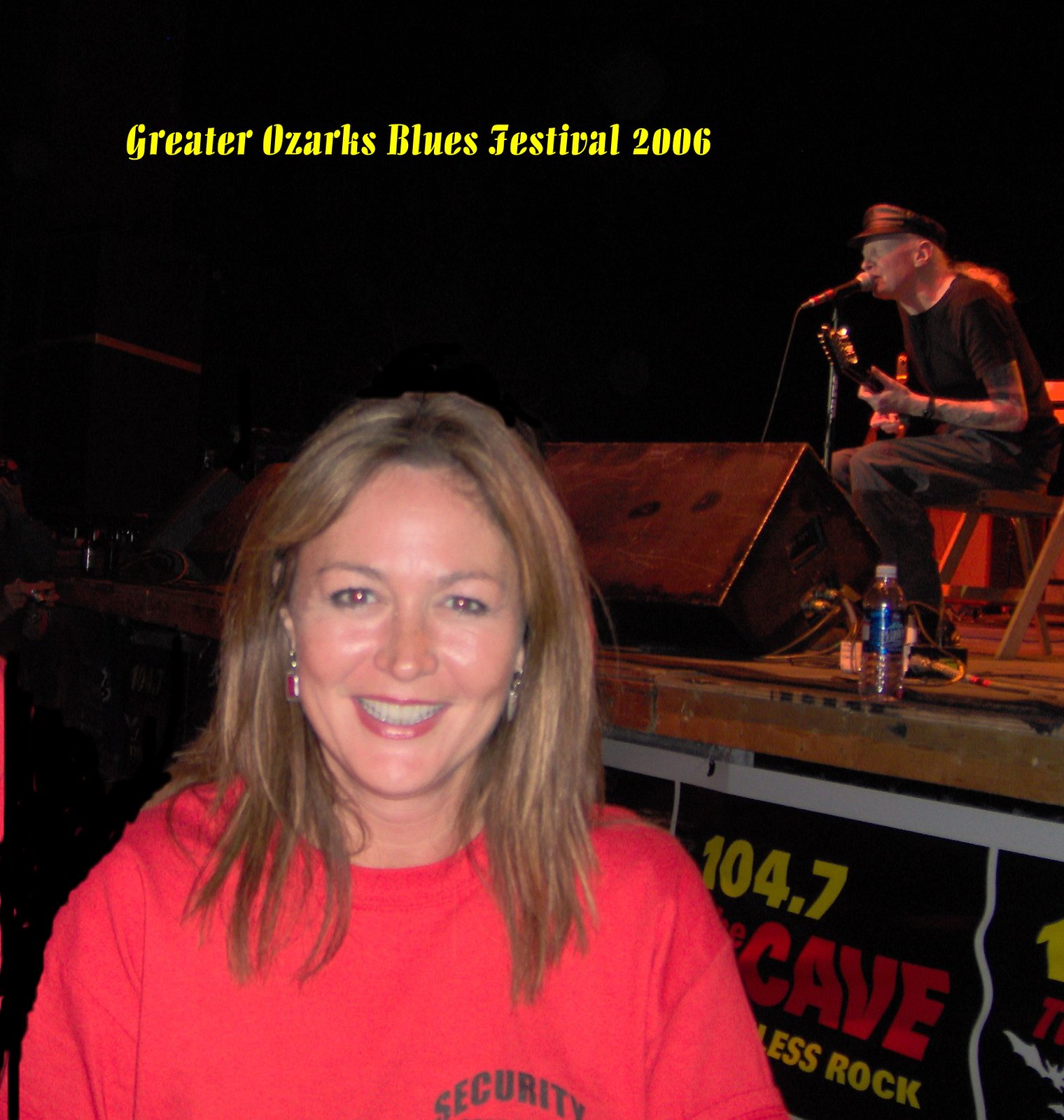In this photograph from the Greater Ozarks Blues Festival in 2006, an attractive young blonde woman stands smiling in front of the camera. She is dressed in a deep pink, possibly red, long-sleeve t-shirt or sweatshirt that says "security" on the right side of her chest, matching her lipstick and coordinating with her pink and silver earrings. Her shoulder-length hair frames her blue or brown eyes. Behind her, the stage is set in a dark environment, likely outdoors at night, with a black backdrop. On stage, an older musician wearing a leather cap, black t-shirt, and gray pants, sits on a wooden folding chair. He is in mid-performance, singing into a microphone with an amplifier for his electric guitar nearby and a bottle of water at his feet. The top of the photo features text in yellow that reads "Greater Ozarks Blues Festival 2006," and a sign with "104.7 The Cave" can be seen at the bottom of the stage.